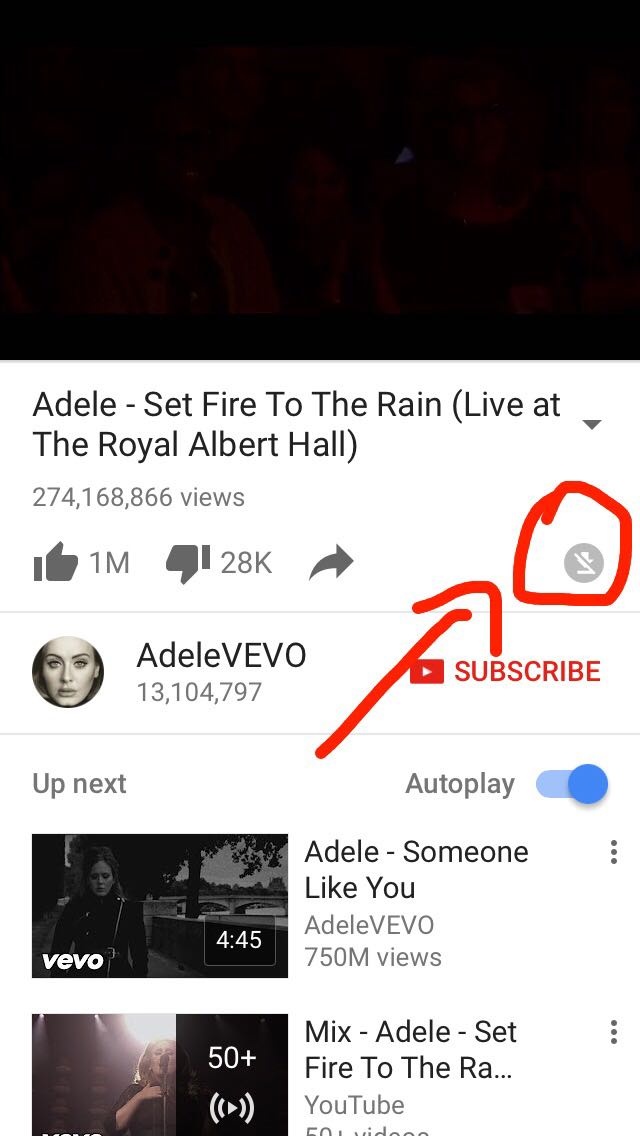Screenshot of a YouTube Video:

This image is a screenshot from YouTube showcasing a video. At the top, there is a dimly lit thumbnail featuring three individuals seated in a dark theater. The image is very dark, making it difficult to distinguish details, but it appears there is a man on the left and two women on the right, all enveloped in a subtle orange hue.

Below the thumbnail, the video title is displayed: "Adele - Set Fire to the Rain [Live at the Royal Albert Hall]." The video has garnered significant attention with 274,168,866 views, 1 million thumbs up, and 28,000 thumbs down. Adjacent to these statistics, a download button is shown, but it is disabled. This button is circled in red, with a hand-drawn red arrow pointing to it from the lower left corner.

Further down, there is a channel button labeled "AdeleVEVO" featuring an image of Adele's face inside a circle. The channel boasts 13,104,797 subscribers. To the right of this is a prominent red "SUBSCRIBE" button, displaying the iconic YouTube logo with its white play triangle set against a red background.

In the "Up Next" section, autoplay is indicated as being on, with the next video being "Adele - Someone Like You" followed by a mix of "Adele - Set Fire to the Rain" along with 50+ other songs.